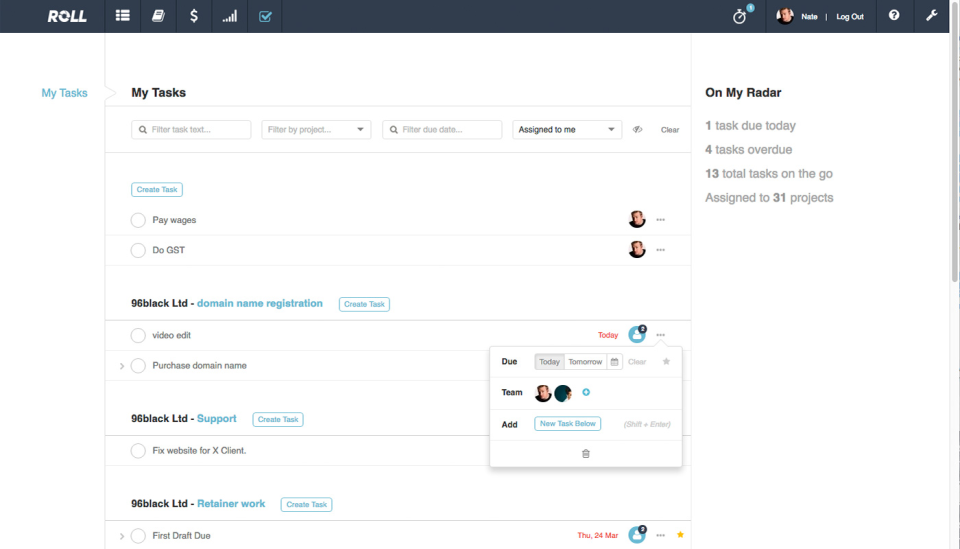The website Roll features a top navigation bar with various icons including a list, a book, a dollar sign, and a bar graph. A user named Nate, a Caucasian male, is signed in, with several unread notifications indicated next to his profile. To the right of his name, there are buttons for logging out, accessing help or support, and a wrench icon likely for settings. 

Currently, the user is within the "My Tasks" section. This area appears to be designed for task management, offering fields such as filter task text, filter by project, and filter by due date. Users can also select options related to pay wages and due GST, hinting at financial functionalities. Nate has already created several tasks that can be toggled on or off, suggesting an integration with a payment platform or comprehensive task tracking.